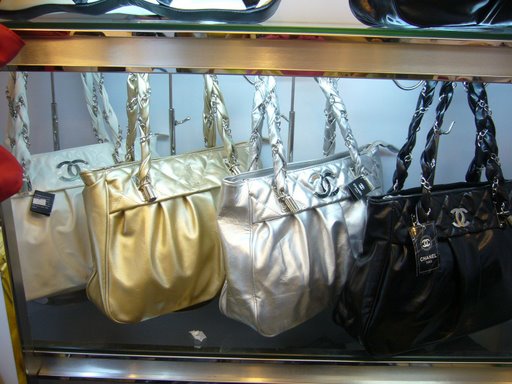The image showcases a collection of four designer handbags hanging in a display case with a glass front and surrounded by a brown wooden frame and a gold barrier. Each handbag features the iconic Chanel logo prominently. Starting from the left, the first handbag is a white bag with a silver Chanel logo in the middle and white braided handles intertwined with silver chains. Next to it is a shiny gold handbag with similar handles. The third bag is a lustrous silver color, also adorned with silver braided handles. Finally, the rightmost bag is a sleek black handbag with a silver Chanel logo in the middle and black braided handles threaded with silver chains, along with a black Chanel tag.